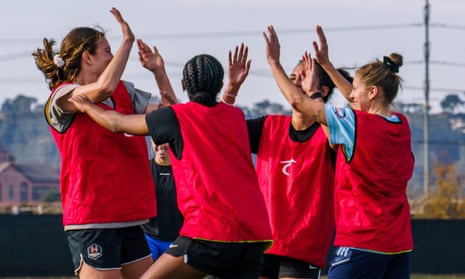The image features a jubilant women's or girls' soccer team, likely celebrating a recent goal or victory. The scene includes at least four or five players, all visibly elated, high-fiving each other in shared excitement. They are dressed in red vests with a small logo, possibly depicting a soccer player, over their standard blue soccer shorts. The team members sport a variety of hairstyles: long braids, a bun, a ponytail, and cornrows. In the backdrop, one can see houses, larger buildings, trees, and power lines, suggesting a community or recreational setting, possibly a practice session given the nature of their attire and overall relaxed demeanor.